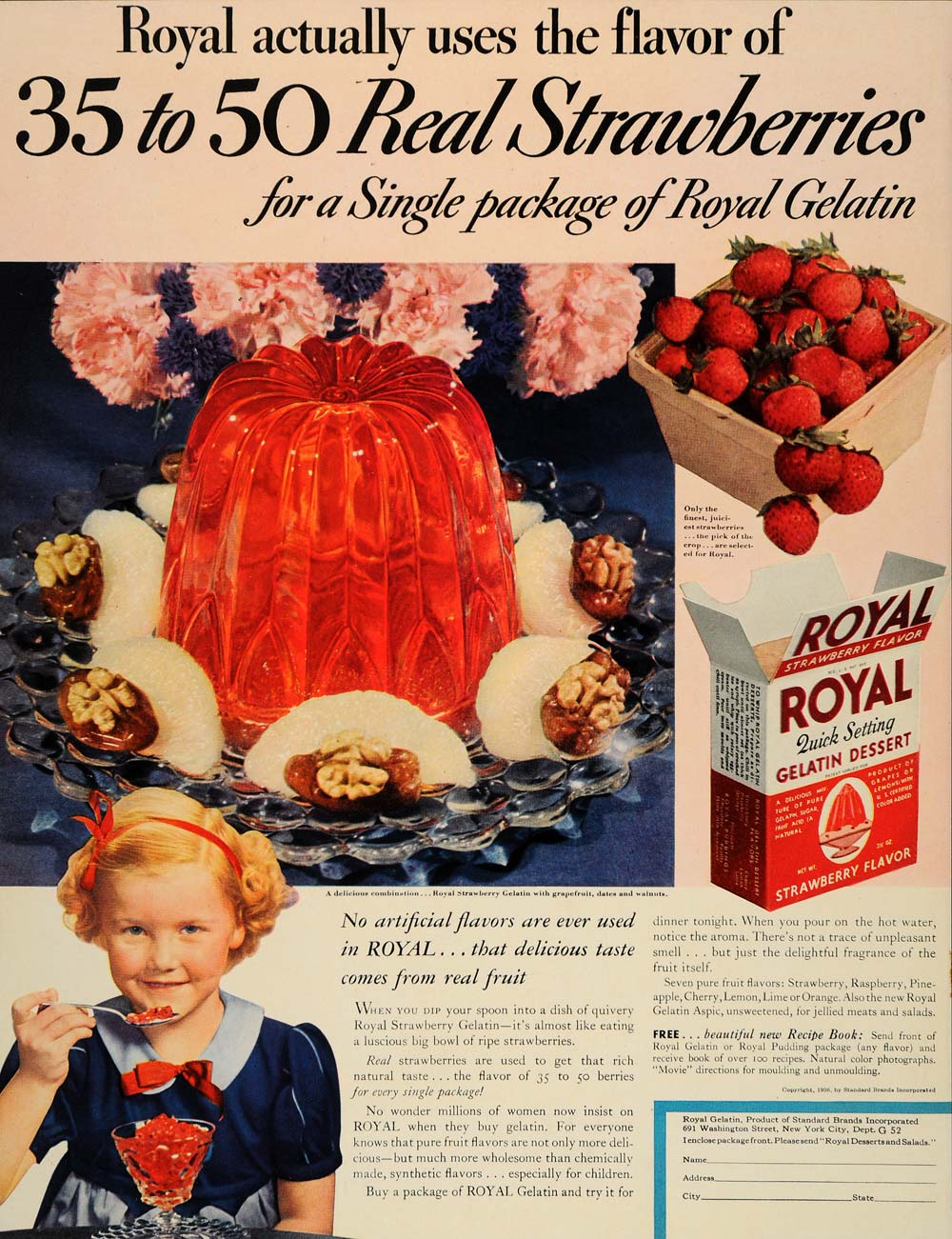This image appears to be a scanned advertisement from an old magazine for Royal Gelatin, specifically highlighting its strawberry-flavored gelatin. The ad boldly states, "Royal actually uses the flavor of 35 to 50 real strawberries for a single package of Royal gelatin." The visual elements include a vibrant image of a gelatin mold, distinctly strawberry-flavored, presented on a glass tray surrounded by chocolates and nuts. Adjacent to the gelatin mold is a box overflowing with fresh strawberries and an open package of the Royal Gelatin mix, emphasizing its rich, authentic flavor. At the bottom of the advertisement, a cheerful young girl with orange hair, adorned with a red bow and dressed in a blue dress, enjoys a bowl of the strawberry-infused gelatin. Additional elements in the ad include various facts about the product and possibly an order form for purchasing the gelatin. The entire composition evokes a nostalgic and appetizing appeal, wrapped around the happiness and delight of enjoying a classic dessert.